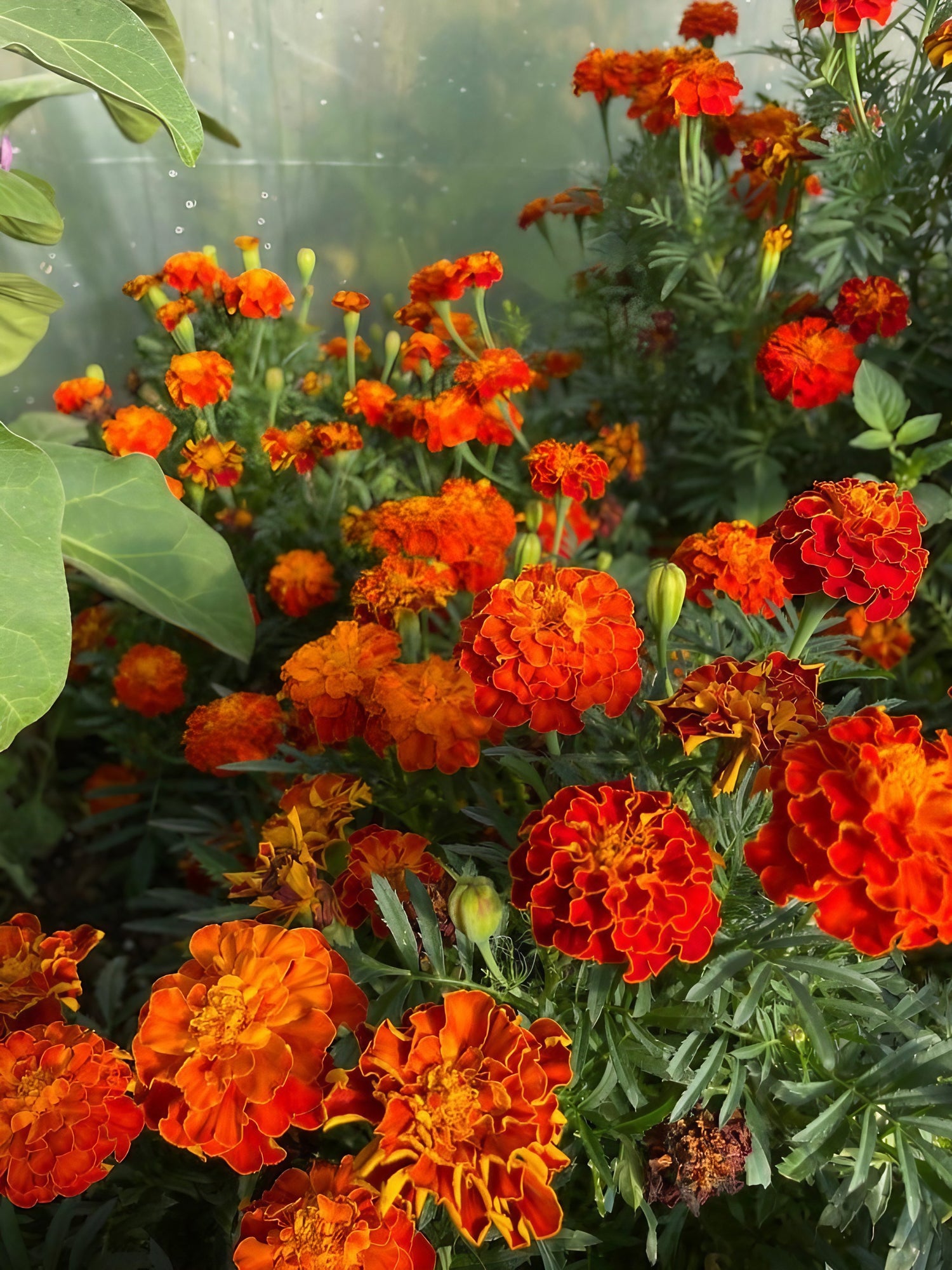This detailed photograph captures a lush array of blooming orange and reddish-orange flowers, known as Ginda flowers in India, flourishing inside what appears to be a greenhouse. The flowers are not sunflowers but present clusters of petals forming rounded shapes at the end of their stalks. Each plant boasts generous knife-like green leaves, some slightly serrated, indicating robust growth. Among the greenery, numerous flowers—approximately 20 to 30—are visible, with some still budding. The background reveals a translucent covering, either glass or tarp, speckled with water droplets, enhancing the greenhouse ambiance. The entire image is saturated with verdant plants and vivid floral blooms, creating a stunning and vibrant horticultural display.